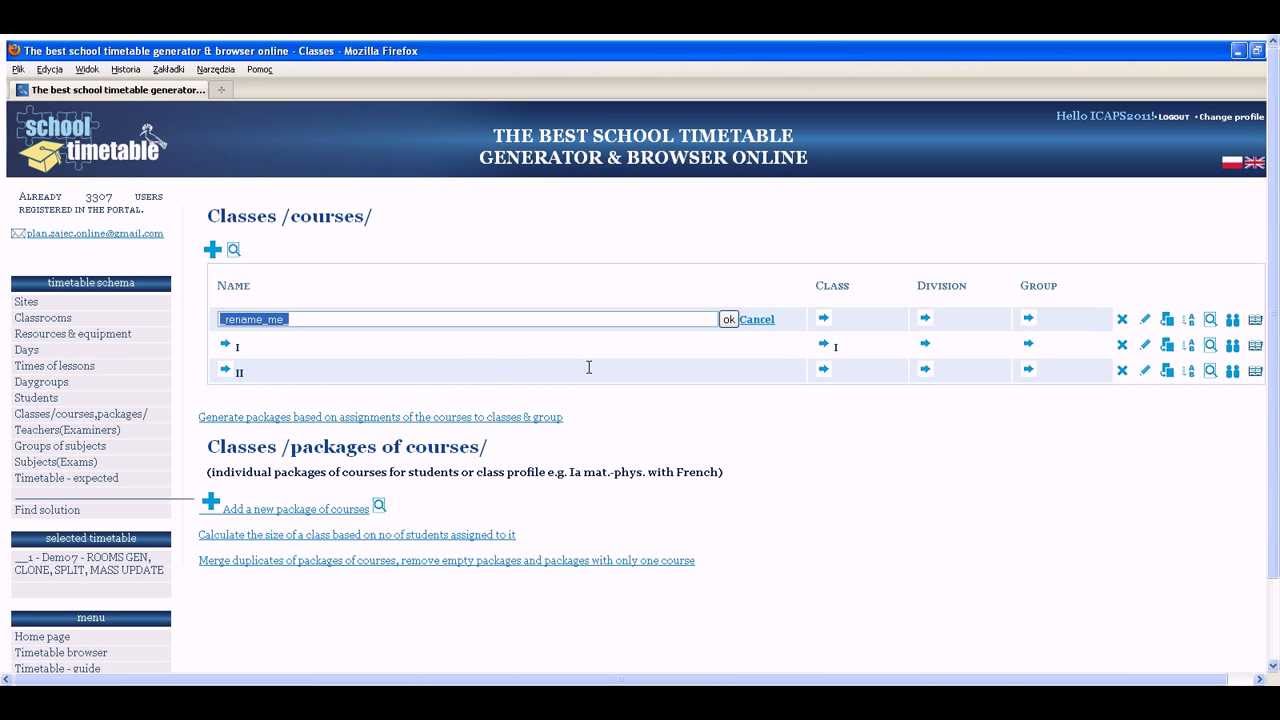This screenshot appears to be an older capture of a website, evident from the design and font style. The image features a blue bar at the top containing the Firefox logo—a stylized, orange fox encircling itself—positioned on the upper left side. The top and bottom of the image are framed by black bars. 

In the main section of the image, there is a light blue bar with a portion of text that reads: "The best school timetable generator and browser online." The logo for Mozilla Firefox is prominently displayed just above this text. On the right-hand side, there are several clickable buttons, along with a white open space.

On the left side of the main content area, there is a darker blue section adjacent to the lighter blue section, which contains text in yellow that reads, "Timetable." The central section reiterates, "The best school timetable generator and browser online."

Additionally, gray-on-gray text is found on the far left side. A white section within the main content area lists categories such as "Classes/Courses." Certain elements in this section are highlighted in blue, with a mixture of white, black, and gray text, rendering some parts hard to read. Towards the bottom, further text indicates "Classes/Packages of Courses," though the smaller font makes it challenging to decipher the rest.

Overall, the image captures a dated interface dedicated to an online timetable generation tool, viewed via the Mozilla Firefox browser.